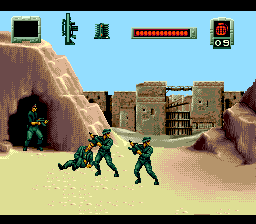A pixelated screenshot from an older video game showcases a military-themed scene. On the left side of the image, there is a pyramid-shaped brown hill with a small cave opening, out of which an armed soldier is emerging, clutching a machine gun. In front of this cave, another soldier lies prone on the ground, possibly injured. Two additional soldiers stand behind him, alert and looking towards the right side of the screen, suggesting an imminent threat from that direction. 

The setting appears to be a fortified area, with walls surrounding the characters, creating a sense of enclosure. At the top of the screen, various weapon icons are displayed, including a briefcase-like item, a formidable rocket launcher, and an unidentified object. Additionally, there is a graphical life meter, indicating the players' remaining health. A grenade icon accompanied by the number '9' signifies the availability of nine grenades for use. This detailed scene captures the intensity and strategic atmosphere typical of classic military video games.